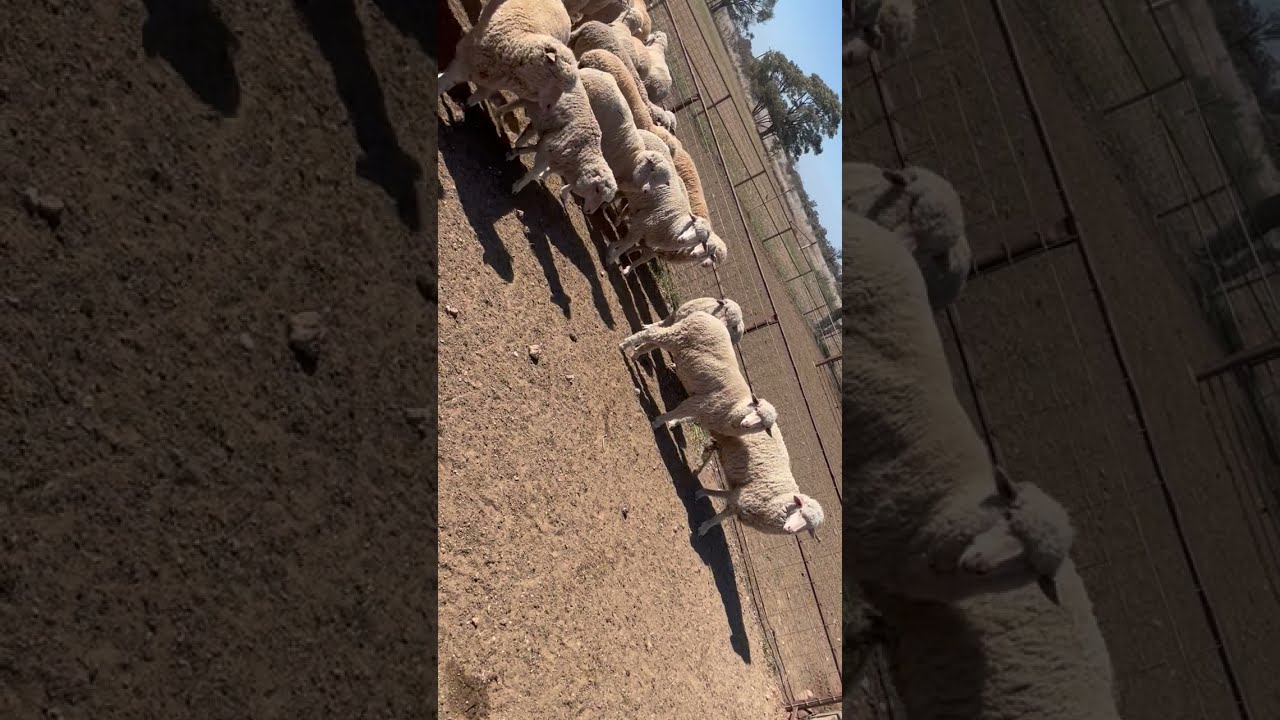This image, rotated 90 degrees to the right, depicts a herd of at least a dozen sheep in an outdoor pen with a dirt-covered ground. The pen is enclosed by metallic fencing that stretches across the scene, from the left to the right, and from the bottom to the top of the rotated photograph. The sheep, with their wool varying from white to light brown and beige, stand in different orientations, some facing the viewer. The setting includes a background of green trees and a bright blue sky, indicating it is daytime. The photograph appears to be part of a composite image; it is laid over larger close-up sections of itself, with these sections flanking the main image on either side. The scene depicts a pastoral environment with the fencing and trees framing the central focus on the sheep.